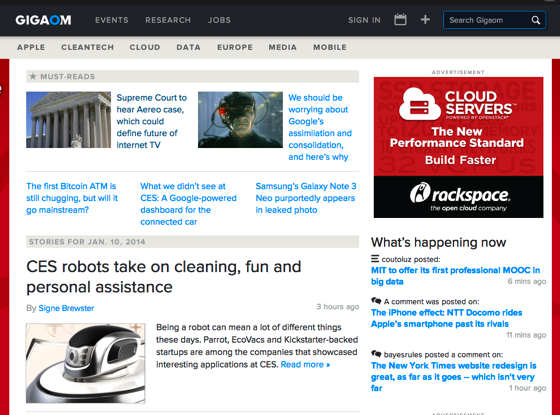The image is a screenshot of the GigaOhm website, a now-defunct online tech publication. The layout of the webpage is wider than it is tall, suggesting it is displayed on a computer screen rather than a mobile device, although it could be viewed on an expanded mobile screen. The GigaOhm logo is located in the upper left corner, with the "O" rendered in blue font while the remaining letters are white. This logo is set against a white background.

Directly below the logo is the main navigation bar, displayed in a black rectangle, with options labeled "Events," "Research," and "Jobs." Beneath this is another navigation bar, this time in a gray rectangle, showcasing various tech-related topics such as "Apple," "Cleantech," "Cloud," "Data," "Europe," "Media," and "Mobile."

The main content area of the page features several articles. Three of these articles are highlighted with images. One article displays a photograph of the Supreme Court building, accompanied by the headline, "Supreme Court to Hear Aereo Case: Could Define Future of Internet TV." Another article features an image of Locutus of Borg from Star Trek: The Next Generation, with the headline, "Why Should We Be Worrying About Google's Assimilation and Consolidation? Here's Why." The articles are dated January 10, 2014, indicating that the screenshot captures content from a decade ago.

Overall, the GigaOhm website screenshot illustrates the publication’s focus on technological advancements and issues, presented in a clean and structured layout conducive to in-depth reading.